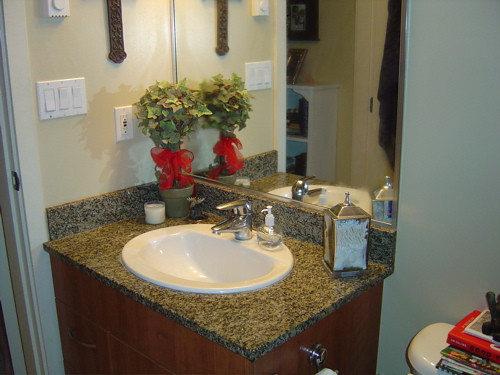The image showcases a well-decorated bathroom with white walls and an array of intricate details. On the top right, there is a white switch and electrical plugs. A wooden wall art piece is mounted above a sleek, silver-framed mirror, which reflects an adjoining room. Within the mirror's reflection, a white wooden desk adorned with framed pictures is visible against a cream-colored wall. A black towel is neatly hung on the door. The bathroom counter features a luxurious marble surface, atop which a white sink and a silver tap are positioned. A vibrant green potted plant, adorned with a red ribbon, adds a touch of nature. Adjacent to the plant is a small, transparent container holding a white candle. Below the counter, brown drawers provide storage space. In the bottom right corner, a toilet seat is visible, with a stack of books in red, green, and white resting on top.